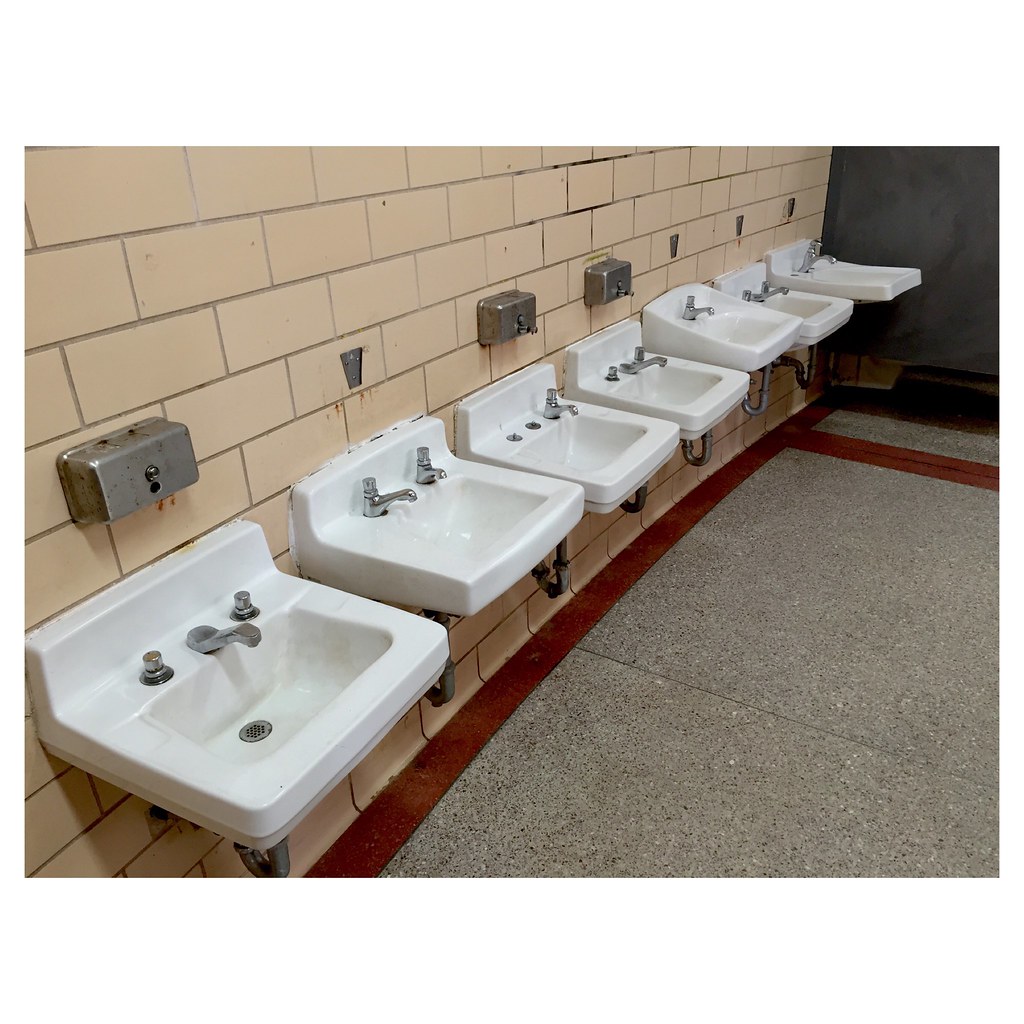The image depicts a worn, older public restroom with a row of seven white ceramic sinks affixed to a grungy, off-white tiled wall. The tiles are brick-shaped, and the grout is stained with mildew and rust marks. Some sinks have a single faucet, while others feature more than one, highlighting their varying shapes and sizes. This hints at a budget or makeshift maintenance style. Above a few sinks, metal paper towel dispensers are visible, while others have only marks on the wall where similar boxes appear to have been removed. The floor has an industrial granite-like appearance with a maroon border and a grainy gray texture that adds to the overall dilapidated feel. A black metal bathroom stall is partially visible in the background, reinforcing the sense of an outdated and unkempt public lavatory.